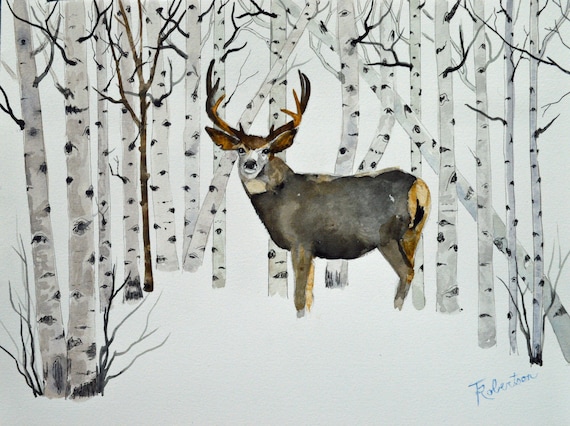In the watercolor painting, a majestic male reindeer, standing upright, is centrally featured in a serene forest scene blanketed with snow. The reindeer's antlers are bold with shades of black and brown, and its body showcases a mix of black, dark grayish, and brown hues. The reindeer's face has a distinctive white area around the nose, with its inner ears also highlighted in brown. The animal's posture suggests it is looking to the side, but with an attentive gaze that meets the viewer's eyes.

Surrounding the reindeer, the forest is composed of slender trees with striking black and white bark, likely birch or aspen, standing leafless in the wintry landscape. The trees frame the scene and extend across the whole background, from left to right. The snowy ground obscures the reindeer's hooves, enhancing the quiet, pristine ambiance of the winter setting. The entire composition is rendered against a white background, lending an ethereal quality to the artwork. In the bottom right corner, the artist's signature, which appears to read "T. Robertson," provides a final personal touch to the painting.